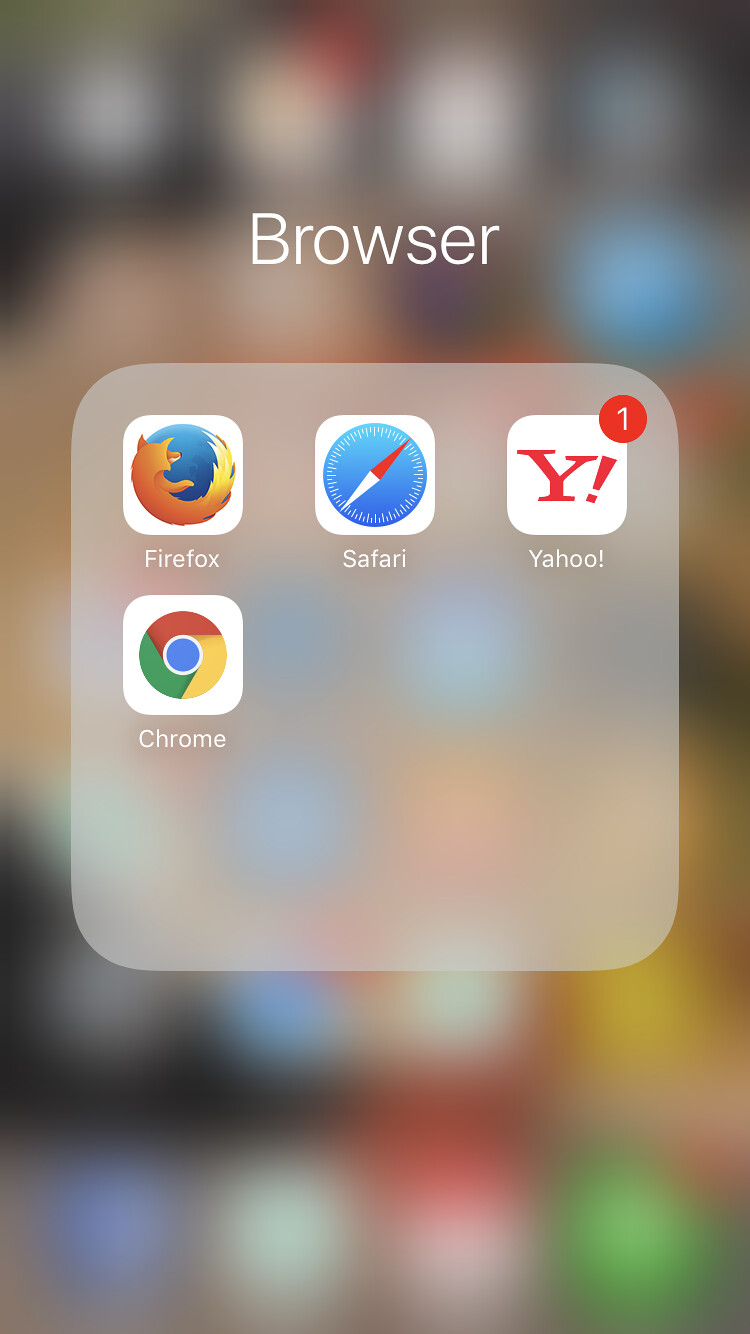The image depicts a portion of a smartphone screen. The blurred background, decorated with a variety of colors such as white, yellow, green, and blue, forms an abstract mosaic behind the primary focus area. At the top of the screen, the word "BROWSER" is prominently displayed in capital white letters. Below this title, there is a light grayish-white rectangular section containing four distinct app icons arranged in two rows. The upper row features Firefox on the left, Safari in the center, and Yahoo, which is marked with a red notification badge displaying the number "1," on the right. Below these, in the second row, is Chrome, standing alone. Each app icon is sharply rendered on a clean white background, making them easily distinguishable.